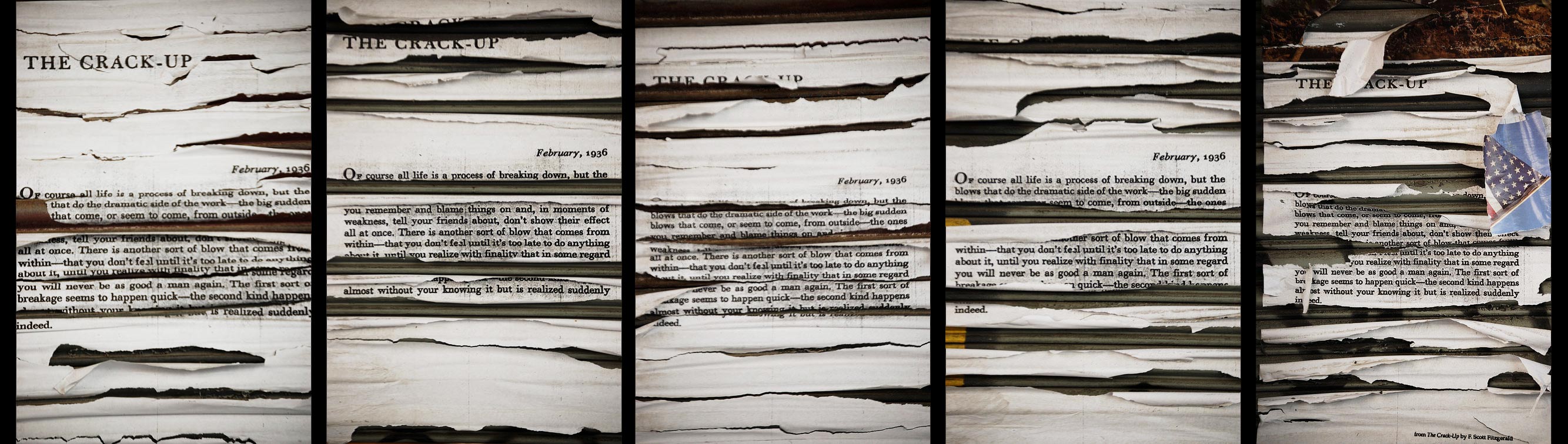The image consists of five squares, each containing a shredded piece of paper that appears to be from the same book. The pages are arranged side by side, and each one has been meticulously pieced back together to attempt to read the content. The text on these pages includes recurring fragments of the title "The Crack-Up." The first square shows the top of the page clearly displaying "The Crack-Up." The second square also shows "The Crack-Up" but has been cut in half. In the third square, only the top letters of "The Crack-Up" are visible. The fourth square offers no visible trace of the title but reveals the date that the letter was written. The fifth square partially shows "The Crack-Up" without revealing the date. All the pages exhibit horizontal slashes, suggesting an almost violent, knife-like mutilation rather than simple tearing.